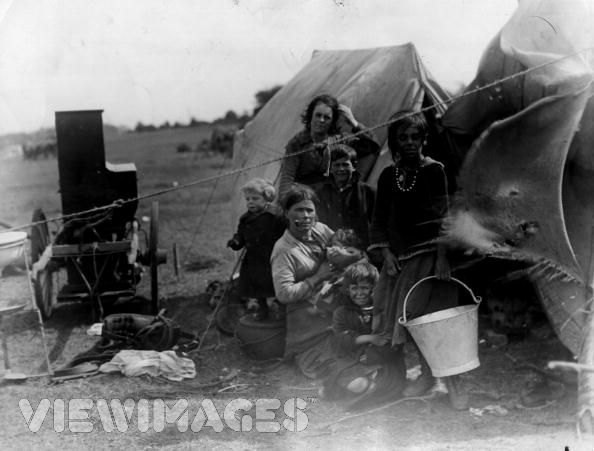This black-and-white photograph, seemingly dating back to the early 1900s or earlier, captures a family scene in front of a group of canvas tents set against a flat plain with a distant hill and a small cluster of trees to the right. A wagon with giant steel wheels can be seen on the left, partially obscuring a stand-up piano. In the foreground, five children and two women are discernible. The woman in the back left holds her hair with her left hand, while another woman, sitting on the ground in the center, cradles what appears to be a baby and has a pipe in her mouth. A young girl in the front right, dressed in a long skirt and black sweater, holds a large metal pail resembling a milk pail. Two boys, one with a black coat and short brown hair and another in a long black coat with short blonde hair, stand nearby. The group is framed by a rope stretched diagonally across the top-right to the middle-left of the image, suggesting it supports the tents. The photograph has a watermark in the bottom left corner that reads, "VIEW IMAGES" in translucent white bubble letters.